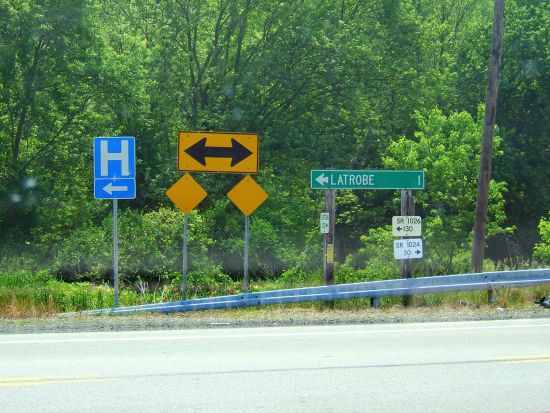The image depicts a highway scene with an adjacent roadway prominently visible in the foreground, characterized by an expansive gray asphalt surface and a lane divider. To the right of the road, a silver guardrail emerges from a gravelly roadside area at an inclined angle. In the background, an abundant array of dense foliage is visible, showcasing a vibrant mix of smaller shrubs and tall trees. A telephone pole can be seen on the right-hand side of the image. 

Several signs are visible along the roadside. There is a blue hospital sign with a left-pointing arrow beneath it. Nearby, a yellow sign features a double-headed arrow pointing in opposite directions, placed above two diamond-shaped yellow caution signs. Additionally, a small green sign supported by two wooden beams indicates "La Trobe" with a left-pointing arrow and states a distance of one mile.